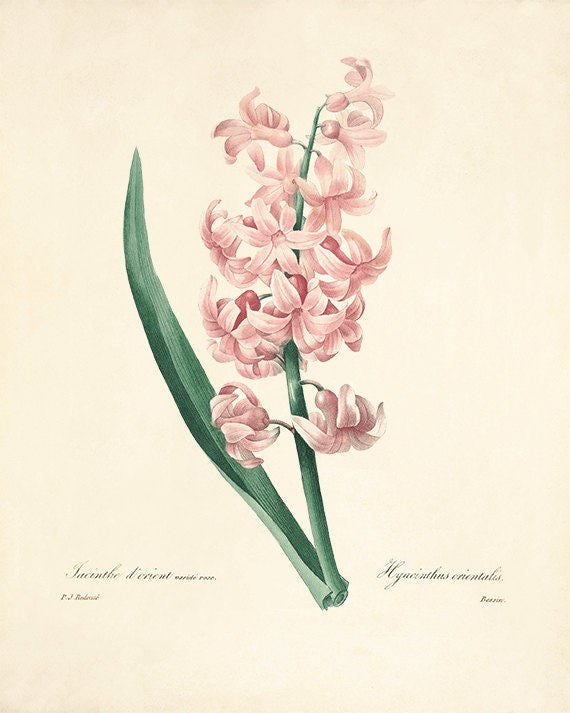This vertical, vintage drawing showcases a meticulously hand-drawn hyacinth flower on a light beige, slightly yellowed, cream-colored background. The illustration features a long green leaf extending from the base of the stout stem on the left side of the flower. The right side of the drawing is dominated by the robust green stem, from which approximately 10 to 20 light and dark pink hyacinth flowers bloom, each detailed with about 6 or 7 petals. The flowers exhibit a blooming appearance, highlighted with careful shading and expert detail suggesting the use of colored pencils. Finishing the aesthetic, cursive black text adorns the bottom of the image, though it is faint and largely unreadable, except for the identifiable word "hyacinth." Overall, the piece reflects the work of a highly skilled artist, capturing the delicate nature of the flowering plant in a timeless, vintage style.